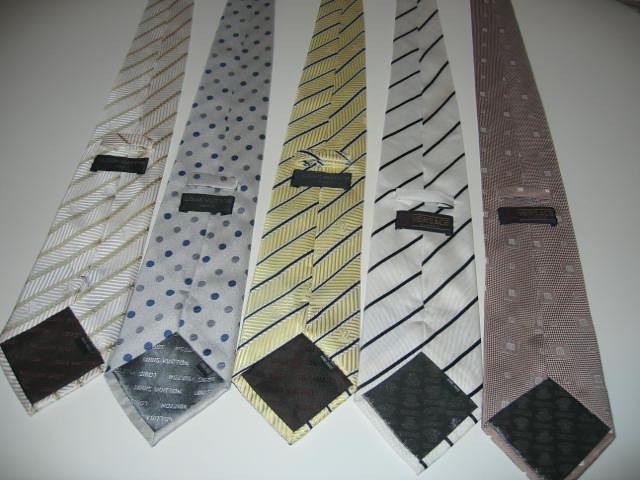The photograph features five neckties laid out on a white surface, possibly a countertop or whiteboard, with their undersides visible. Each tie is displayed with its wider end facing the viewer. From left to right, the ties are as follows: the first tie is beige with darker beige diagonal stripes; the second tie is gray adorned with blue and gray polka dots; the third tie is gold with diagonal blue stripes; the fourth tie is white with black stripes in a diagonal pattern; and the fifth tie is a reddish-brown hue with small square designs. The visible black squares on the underside of each tie indicate the areas where the brand labels are typically attached, highlighting the ties' reverse sides.